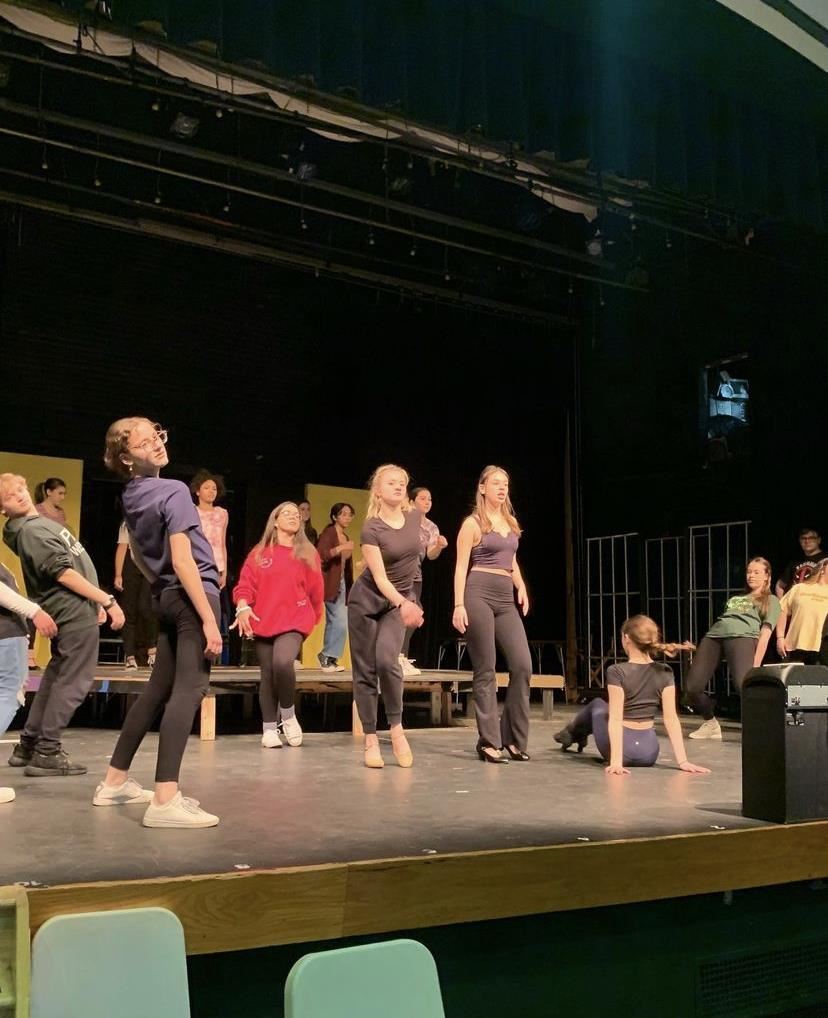This realistic photograph, oriented vertically in a slightly angled shot, captures a high school dance rehearsal or play practice on a stage. The scene comprises about 10 to 12 teenagers, mostly white, with a few individuals who might be black or Asian. The majority are female, wearing casual attire—primarily black or blue yoga pants paired with tank tops, while a notable few sport distinct colored clothing, such as one person in a red sweatshirt and another in a green one.

The stage, viewed from slightly off to the left, features a distinctive light-colored wooden strip running across its front, with a gray cement-colored surface. In the bottom left of the image, two light green chairbacks or pieces of plastic are visible, possibly part of the auditorium seating. The dancers are positioned with some facing each other from opposite sides of the stage, often bent backward or swaying, suggesting a choreographed routine. Three individuals in front are either walking or engaged in a dance motion, while others in the back occupy a higher level of the stage.

Above, the stage remains unlit with visible scaffolding and regular overhead lights, emphasizing that this is a rehearsal rather than a fully staged performance. The environment appears to be a gymnasium or auditorium, as inferred from the surroundings and setup.